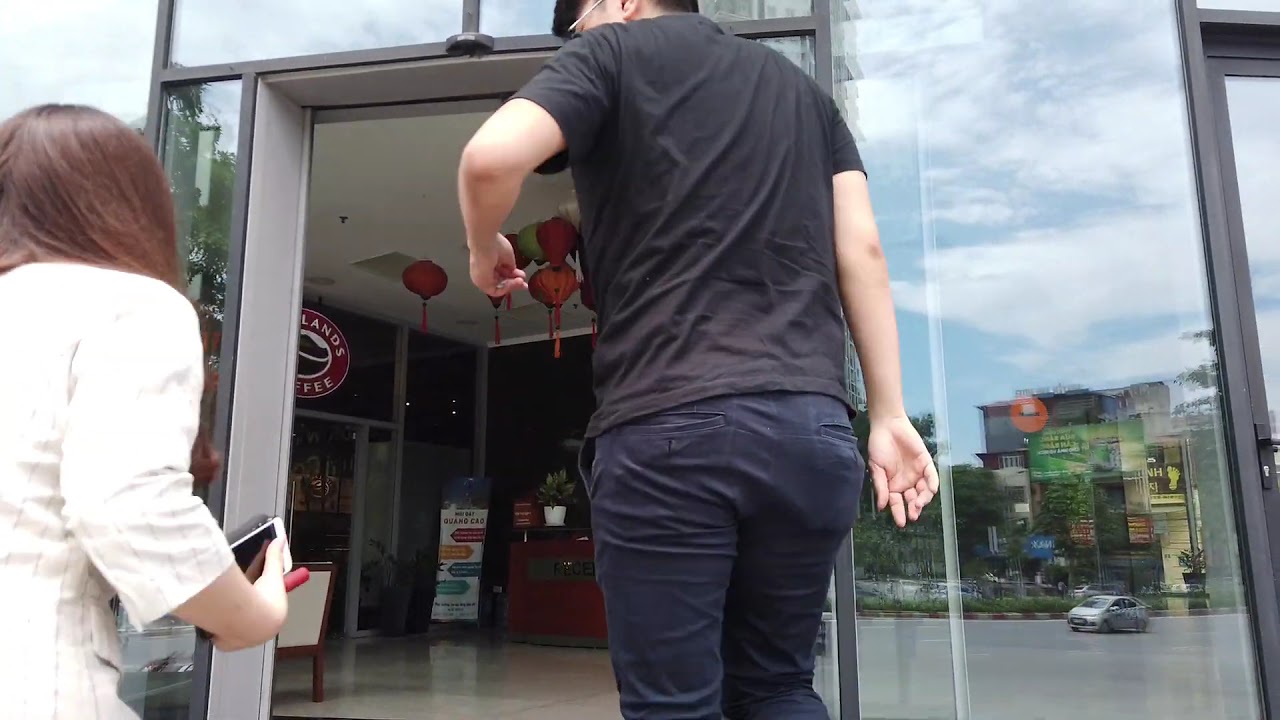The photograph captures the exterior of a building with an open glass gate, revealing the interior and hinting at a business-like setting, possibly a store or mall. In the foreground, two people walk towards the entrance with their backs to the camera. On the right, a man in a black t-shirt, blue jeans, and wearing glasses strides with his arms positioned asymmetrically; his right arm is relaxed by his side, while his left is raised. To his left is a woman wearing a white quarter-length sleeve shirt, brown hair falling past her shoulders, and holding a phone in her right hand. The woman appears lower than the man, suggesting she might be on a step or incline, rather than height difference. Inside the building, the floor is lined with cream-colored tiles and the ceiling is adorned with hanging decorations. Through the glass walls surrounding the gate, reflections reveal an urban backdrop with cityscape elements, including tall buildings and street scenes. Additionally, to the left inside, there’s a business identified as "Something Lands Coffee" with a distinctive red logo above its glass door.